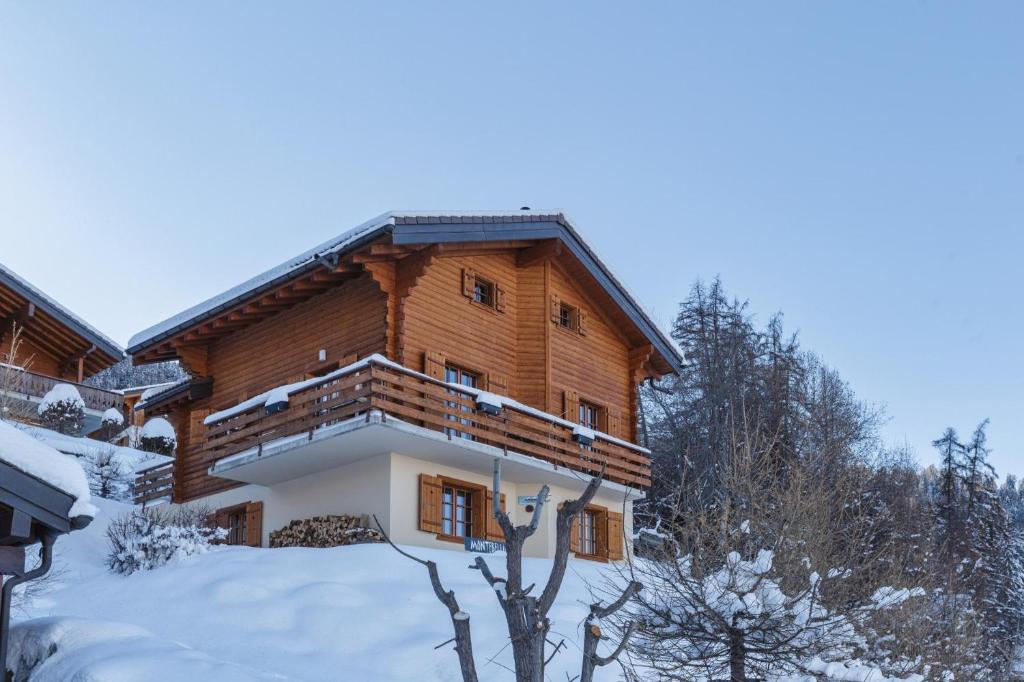This image captures a three-story house resembling a log cabin, set in a serene, snowy landscape. The house’s exterior features wooden upper floors with a metal, triangular roof designed for snow runoff, and a cream-colored ground floor with wood-framed windows and shutters. A wraparound deck extends from the second floor, encircled by a snowy yard adorned with barren trees bearing no foliage. The scene is bathed in brilliant sunlight under a rich, cloudless blue sky, emphasizing the crisp, cold winter day. Snow blankets the ground, the house’s roof, and the surrounding trees, while a snowbank with partially covered bushes lines the base of the house. There are no people or additional text in the photograph, allowing the natural beauty and the quiet, wintry setting of the cabin to stand out prominently.